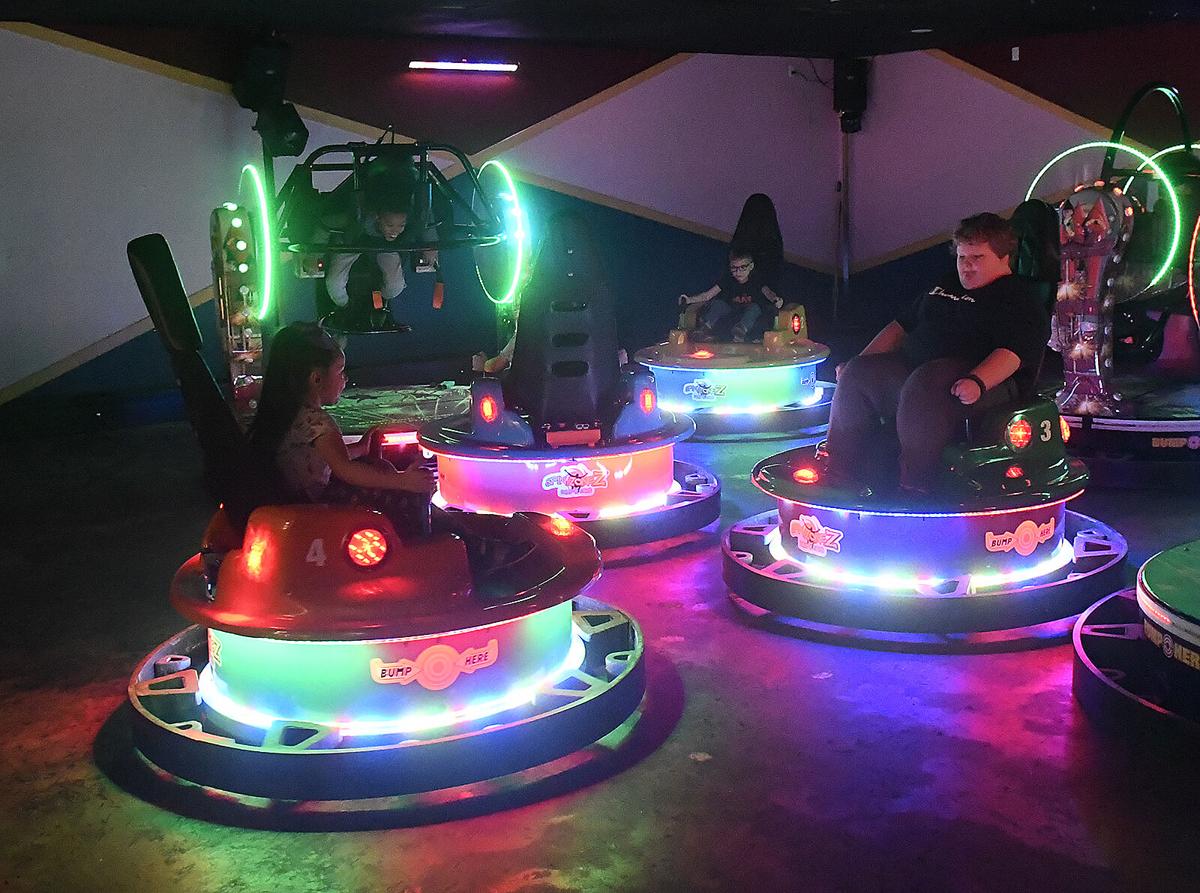In this vibrant and colorful image, four children are engaged in the thrill of bumper cars. The room is brightly lit with a dazzling array of neon lights. Each bumper car is distinct in color and emits a soft glow from their circular bases, enhancing the playful atmosphere. We observe three boys and one girl immersed in the fun. The girl, positioned on the left, rides a cart numbered 4, wearing a white blouse and pants, while the boy on the right maneuvers a cart labeled with the number 3, dressed in a black t-shirt and gray pants.

The bumper cars are not the traditional kind; rather, they feature a unique circular design and come with high back supports for safety during collisions. The neon lighting under the cars and scattered throughout the room creates a vivid spectacle of colors—primarily light blue, white, red, green, and orange—further animating the setting. A boy in a green cart is seen readying to ram the girl, accentuating the playful chaos of the moment. Meanwhile, in the background, another boy with a t-shirt and blue jeans appears eager to join the action. Intriguingly, a figure resembling a boy seems to hang from the wall on the left side, adding to the dynamic and energetic ambiance of the carnival-like space.